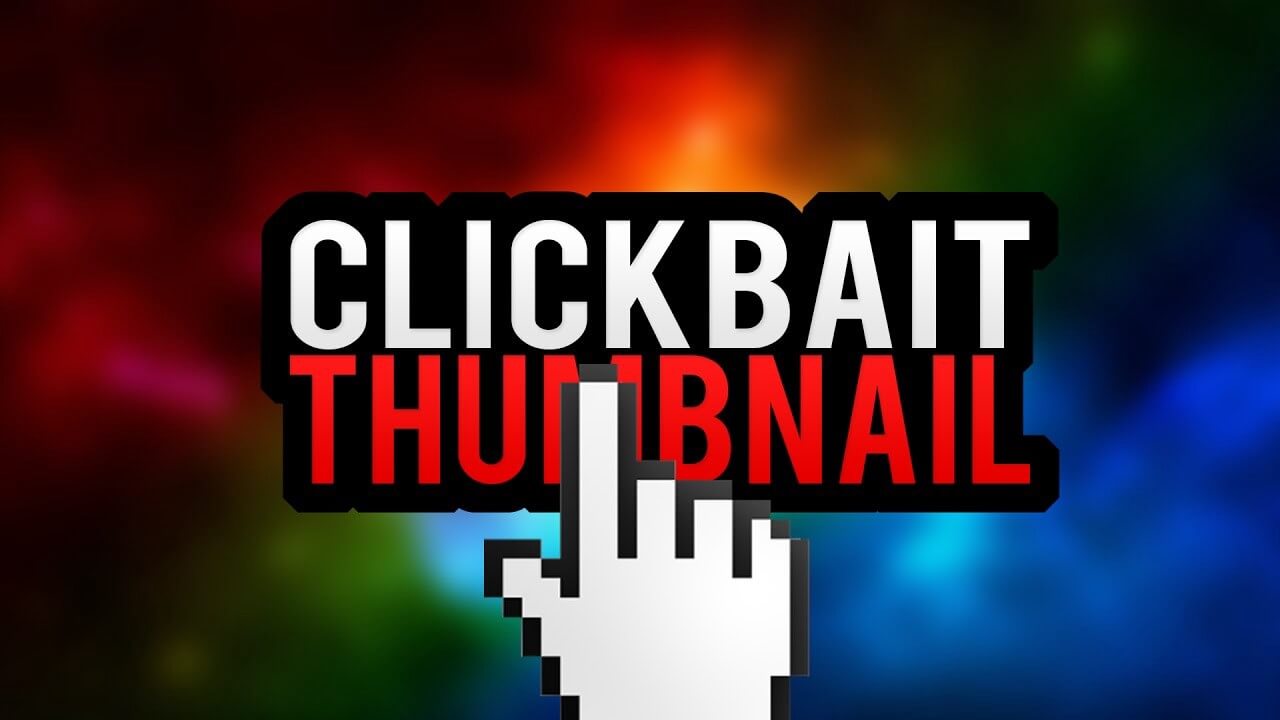The digitally produced horizontal rectangular website image features a vibrant, abstract background with an explosion of colors including deep reds, purples, oranges, yellows, greens, and varying shades of blue. A pixelated hand, with its index finger pointing upright and thumb extended, is prominently positioned over the background, partially obscuring the last letter of the word "thumbnail." The text, arranged horizontally in the center of the image, reads "clickbait" in white and "thumbnail" in red. The chaotic, multicolored background, reminiscent of a rainbow with an added lens flare effect, adds to the playful, comedic style, suggesting a stereotypical clickbait image.